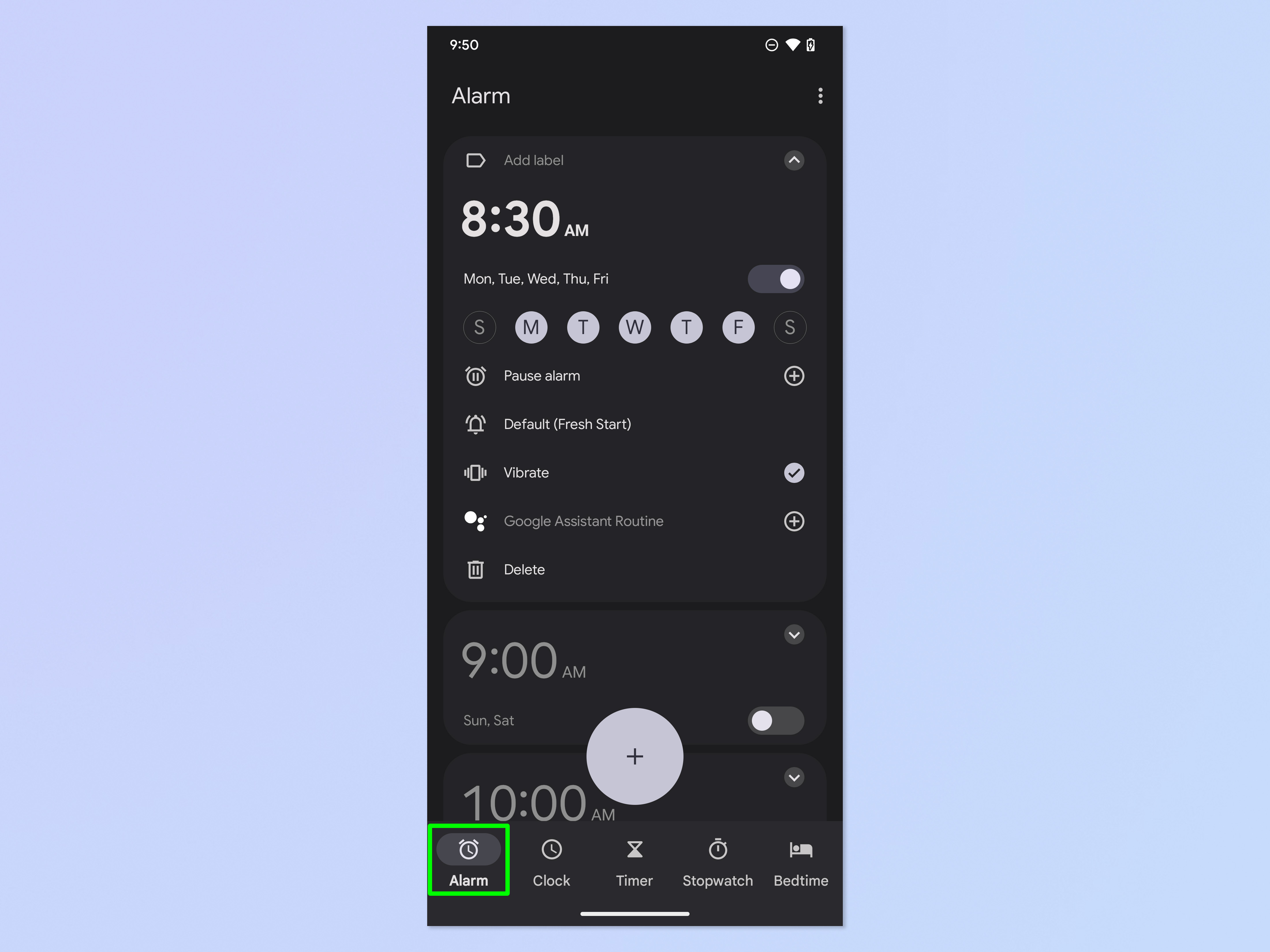The image features a device screen, likely a smartphone or tablet, against a light grayish-purple background. At the top left corner of the screen, the time is displayed as 9:50, accompanied by the "Do Not Disturb" icon on the right. Signal strength indicators and a charging battery icon (less than half full) are visible, with the word "alarm" on the left and a vertical three-dot menu icon on the right.

Below this, there is a dropdown menu with "Add label" and an upwards arrow on the right side. The main interface displays two alarms. The first alarm is set for 8:30 AM on weekdays (Monday to Friday), and appears to be toggled on, indicated by the white background of the day initials (MTWTF), while the initials for Sunday (S) and Saturday (S) are black.

Additional options include:
- "Pause alarm"
- "Default"
- "Fresh start" (with a checkbox indicating it is selected)
- "Google Assistant routine" with a plus sign to its right
- "Delete"

Below that, there is a second alarm set for 9:00 AM on weekends (Saturday and Sunday), also seemingly toggled on, though the distinction of the toggle states (white circle) is unclear.

Overlaying the screen content is a white circle with a plus sign in its center, likely indicating an option to add a new alarm.